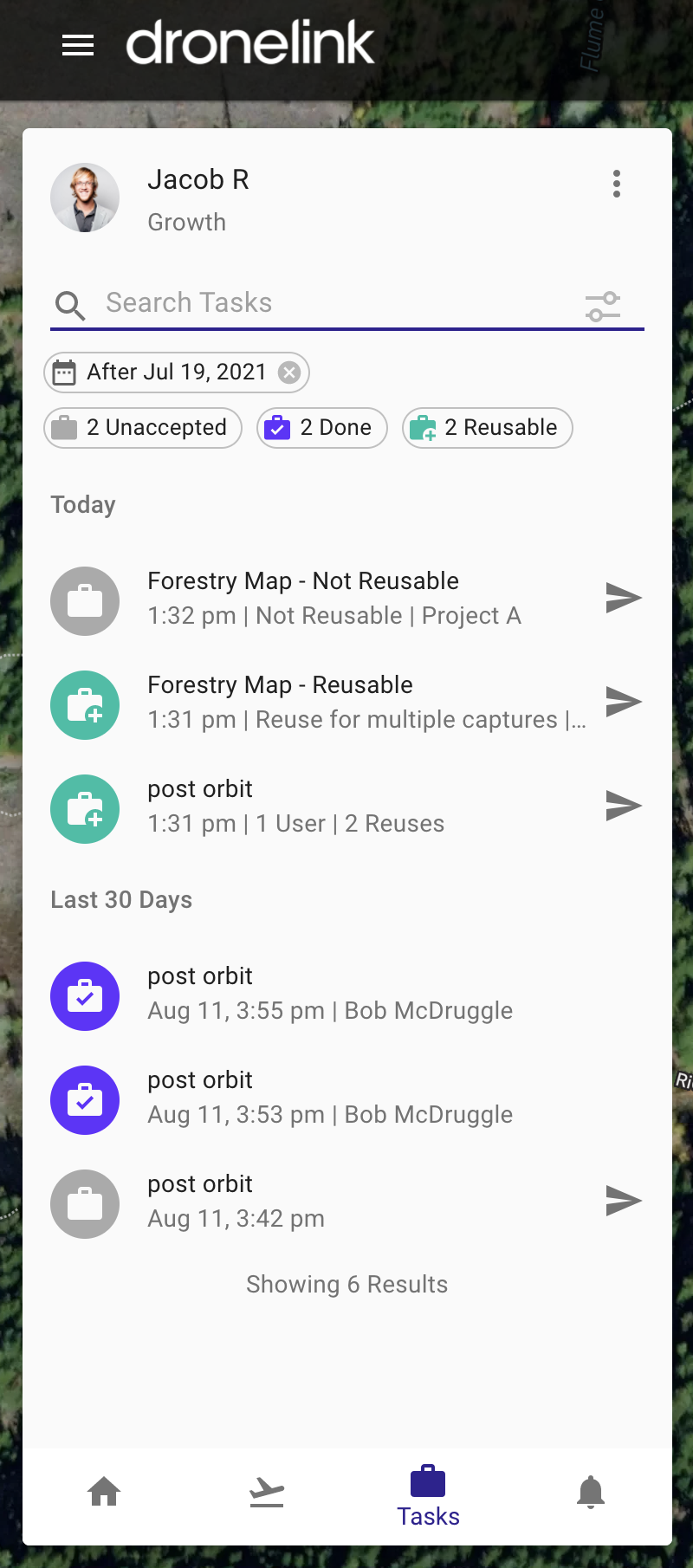This image is a screenshot from a mobile phone, vertically oriented. At the very top, there is a black bar with "DroneLink" written in white text and a menu icon on the top left corner. The background of the image is somewhat unclear but seems to depict green foliage and possibly a grayish stone path or something similar.

In the center of the screen, there's a vertical gray box displaying the name "Jacob R. Growth" along with a profile picture of a man. The man appears to be blonde with a gray background, wearing a gray sweater over a dark green shirt. Below the name and profile picture, there is a search bar labeled "Search Tasks."

Further down, there is a calendar icon button indicating a date: "After July 19th, 2021." Beneath this, there are three status indicators: "2 Unaccepted," "2 Done," and "2 Reusable."

The next section is labeled "Today" and lists several tasks related to a forestry map project. 
- At 1:32 PM, there is a non-reusable forestry map task.
- At 1:31 PM, there is another forestry map task that is marked reusable.
- At 1:31 PM, a task description indicates "Reuse for multiple captures Post-Orbit."
- Post-Orbit-related tasks are listed for August 11th at 3:55 PM and 3:53 PM, both associated with "Bob McDruggle."
- Another Post-Orbit task by "Bob McDruggle" at 3:42 PM on the same date.

Finally, the bottom of the image shows the text "Showing 6 results," summarizing the listed tasks.